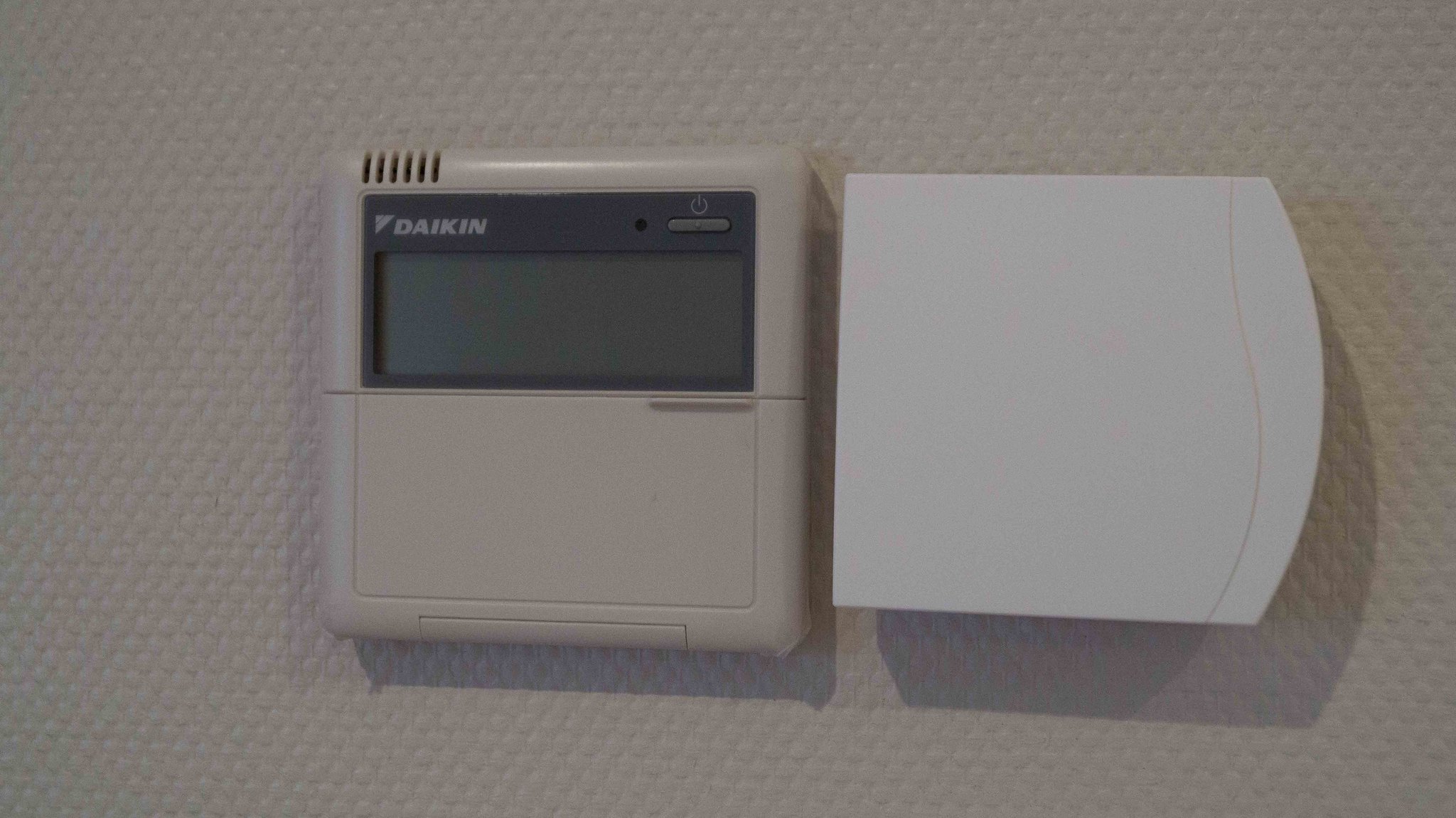The image features two wall-mounted devices against a tan, textured wall. 

On the left is a tan-colored device that appears to be some type of alarm system, potentially for carbon monoxide detection. This device is square-shaped with vents in the upper left corner, likely indicating the presence of a speaker. A digital screen, currently inactive with no visible letters or numbers, occupies the center of the device. At the bottom, there is a finger plate for opening a door, although the door is currently closed. The brand name "Daikin" is displayed in the top left corner, and a power button, marked with a power symbol, is situated in the top right.

On the right is a white, square device with a slightly oval right side, giving it an arch-like appearance. This device has a closed door on it, concealing its purpose. The exact nature of this device is unclear.

Both devices are securely mounted on the rough-textured, tan-painted wall, highlighting their functional and purposeful presence.